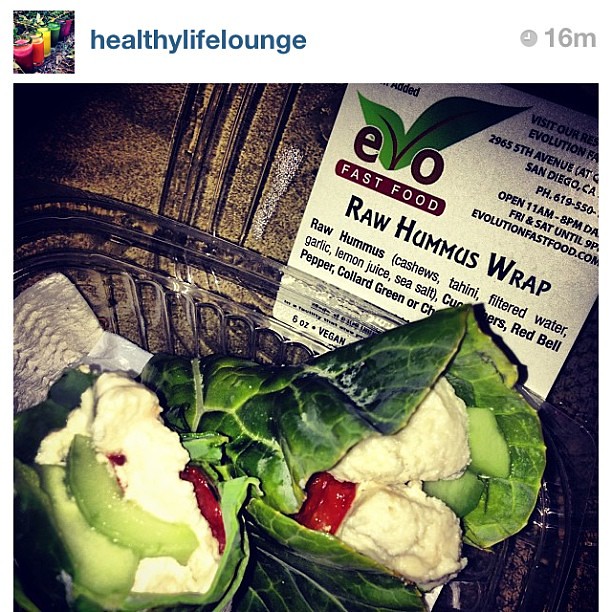The image appears to be a large square photo, likely taken from a social media account associated with Healthy Life Lounge, as indicated by the blue text and small square profile picture in the upper left corner. To the right, a clock icon indicates the image was posted 16 minutes ago.

The main focus of the image is a glass dish containing large lettuce wraps, specifically advertised as "Raw Hummus Wrap." This is confirmed by a detailed white sign behind the dish. The sign is labeled "EO Fast Food" in the upper left corner, decorated with leaf images, and provides address and telephone information in the upper right corner. The main text on the card boldly states "Raw Hummus Wrap" and lists its ingredients: raw hummus (made with cashews, tahini, filtered water, garlic, lemon juice, sea salt), cucumbers, red bell peppers, and collard greens. The glass dish, positioned centrally and slightly to the lower left, contains several of these substantial lettuce wraps, neatly illustrating the plant-based, raw food offering from EO Fast Food.